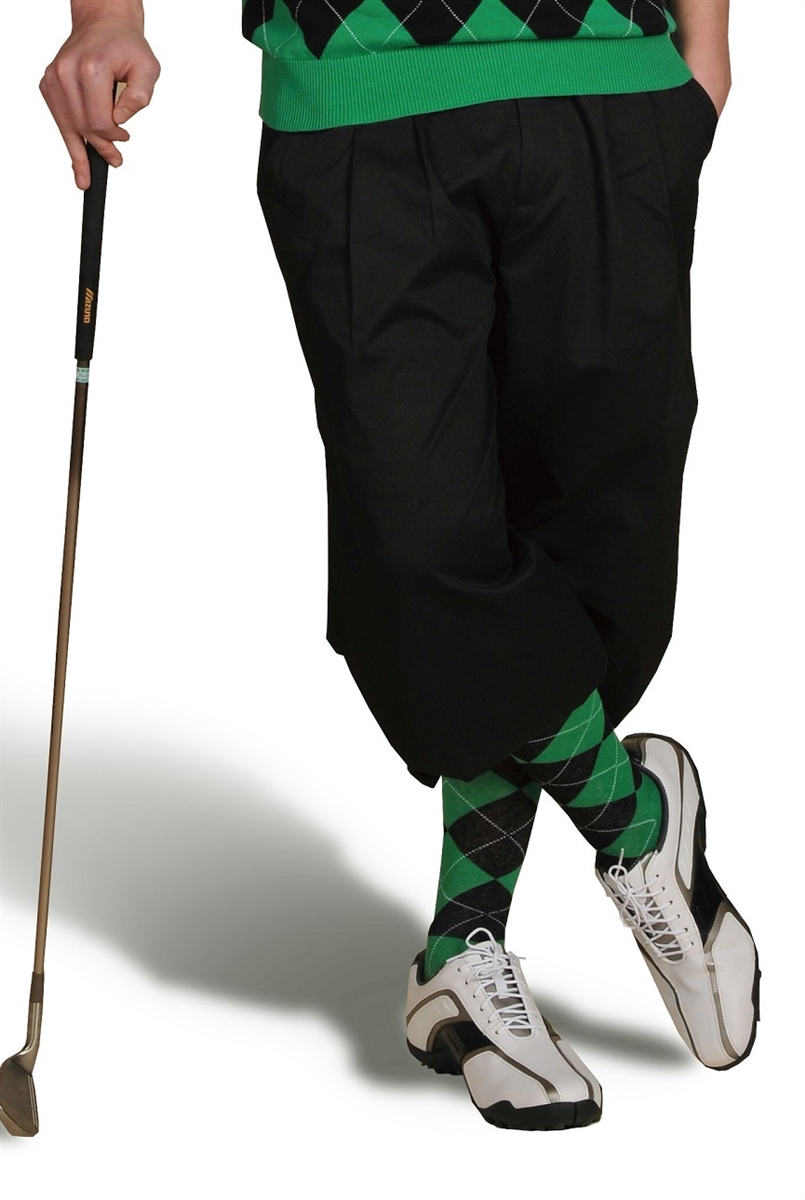This vertically rectangular, full-color photograph, likely taken by a professional indoors under artificial light, features a posed shot of a Caucasian individual wearing a vintage golf outfit, evocative of Payne Stewart’s style. The subject is pictured from just above the waist down against a stark white background with a shadow cutting off sharply. The individual's gender is undetermined due to the image’s focus being primarily on the clothing and pose.

He is dressed in a green sweater with black checkered patterns that match his knee-high socks. The black pleated knicker-style pants end just below the knee, giving a clear view of the matching socks. He wears classic white golf shoes adorned with a black streak. The subject's left hand is casually placed in his pocket while his right hand, which is slightly bent at the wrist and extends out of the frame, grips a putter with a black handle resting on the ground. The stance exudes a leisurely yet poised demeanor, with his left leg crossed over the right foot, toe touching the surface, as though he is waiting for his turn to putt. The only other element in the image is the shadow extending from his feet to the left, contributing a subtle depth to the otherwise minimalistic background.